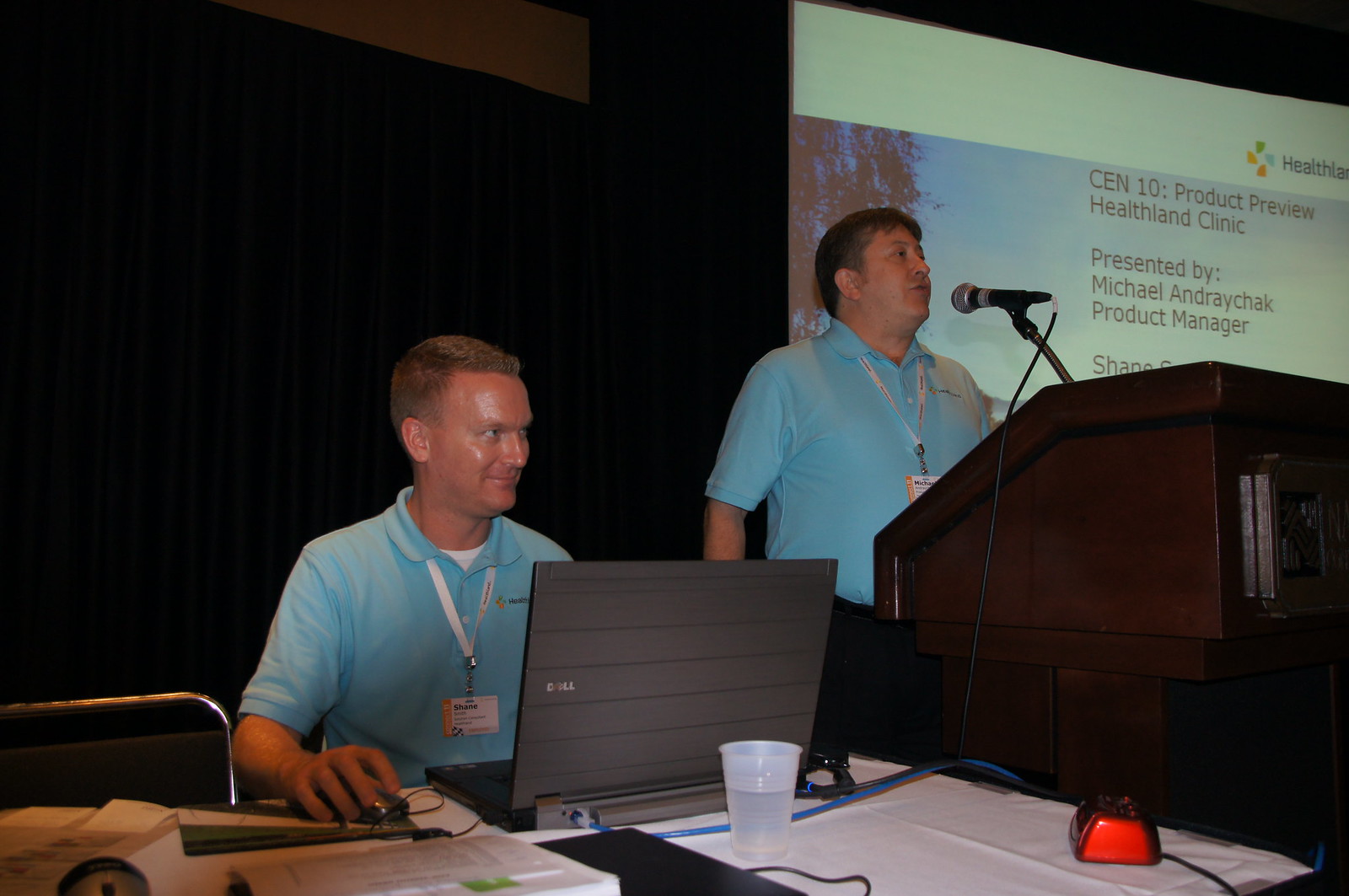The image captures two men delivering a presentation on health. The man on the right is standing behind a podium, speaking into a microphone. He is wearing a blue shirt with a lanyard that has a card attached to it, and has darker hair. Directly to his left, another man, also wearing a blue shirt with a lanyard, is seated in front of a laptop, with his hand on a mouse. He is smiling and looking towards someone in the audience. Both men appear to be from the same organization, likely indicating their shared involvement in the presentation.

Behind them is a large projector screen displaying a slide that partially reads, "Send 10 product preview health land clinic presented by Michael Erichuk and product manager," though the full text is cut off. The background surrounding the stage is black, making it difficult to discern additional details.

The table in front of them is cluttered with various items, including paperwork, a cup of water, a red box, and several wires, suggesting an active and possibly impromptu setup for their presentation. Both men are engaged with their audience, highlighting the interactive nature of their session.